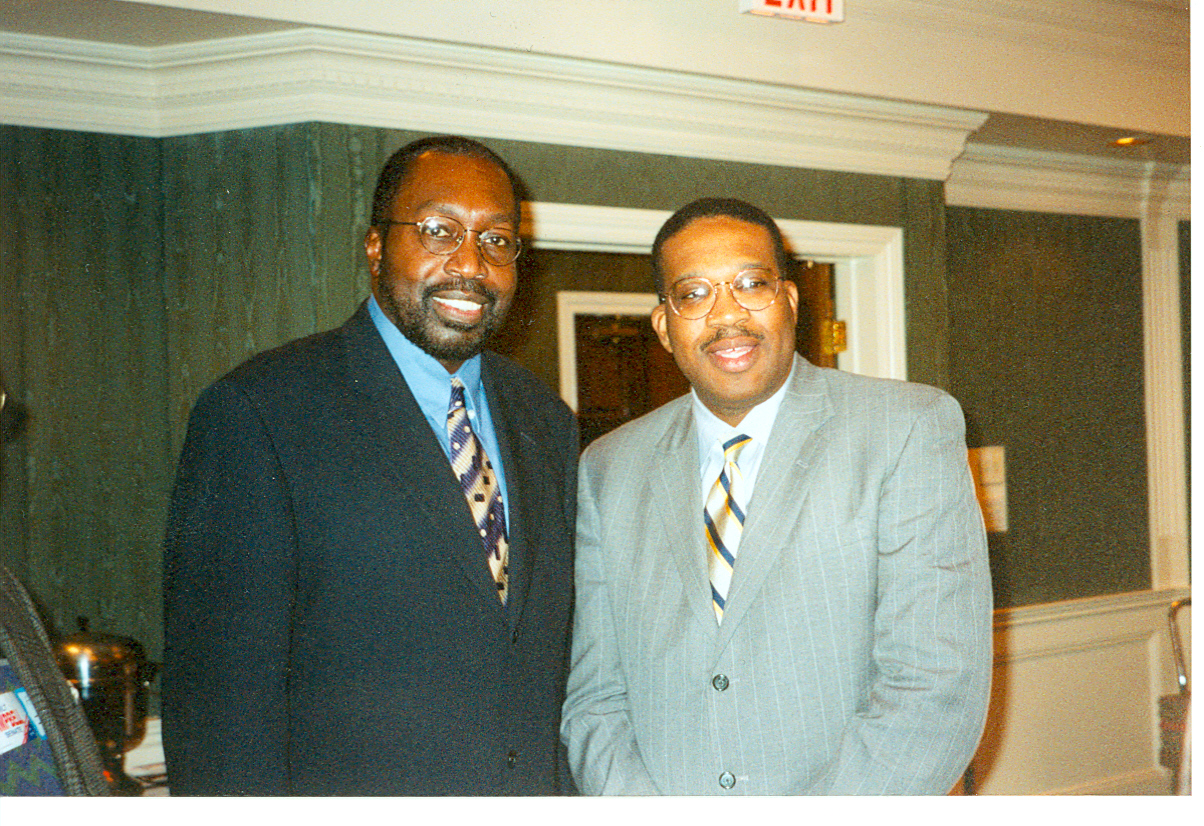In this image, two men with dark skin are smiling at the camera inside a public building. The background features a greenish wallpaper with white panels above and below, and the barely visible edge of an emergency exit sign at the top. There are indistinct objects on the sides, and the door behind them is partially obscured by their bodies. 

The man on the left appears older, possibly in his 40s or early 50s, with darker skin. He has short hair, a full beard, and wears thin-rimmed eyeglasses. He is dressed in a dark blue suit jacket, a light blue shirt, and a blue-and-yellow striped tie with little black and white abstract shapes.

The man on the right, likely in his 30s, has lighter skin. He also has short hair but only a mustache, and he wears thin-rimmed eyeglasses. His attire includes a gray pinstripe suit with a white shirt and a gold tie featuring blue stripes. Both men have amicable expressions and are the main focus of the photograph.